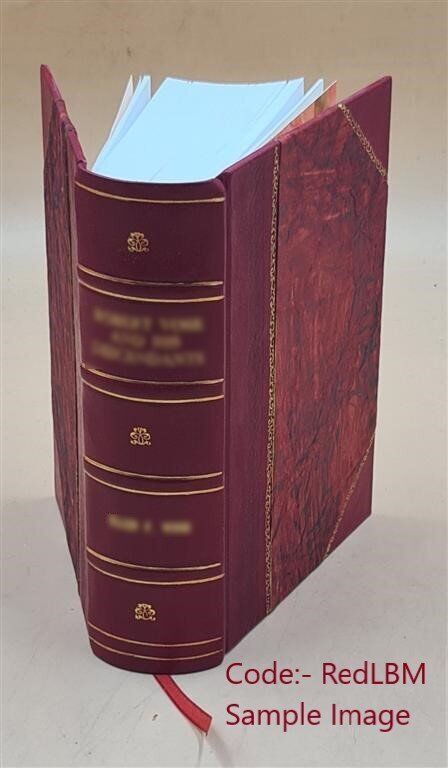The image shows a thick, ornate book with a cherry red cover and white pages, evoking the feel of an old-style encyclopedia or a Bible. The spine of the book features gold threading, though the text is intentionally blurred and illegible. The book stands upright, with light blue-edged pages fanning open and a red tag bookmark hanging from beneath it. At the bottom right-hand corner of the image, there is a text label reading "Code RED LBM," followed by "Sample Image."